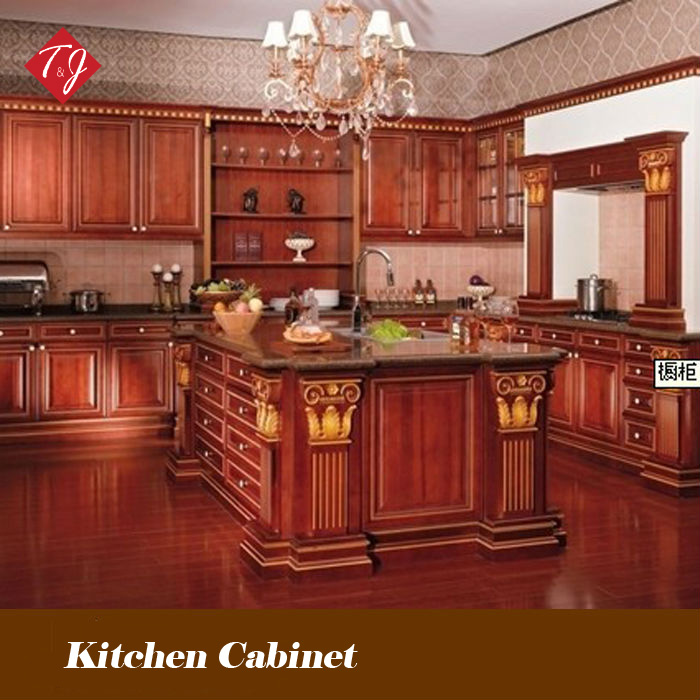This image depicts a spacious and elegantly designed kitchen, primarily constructed from dark reddish-brown stained wood, lending it a warm and sophisticated ambiance. The kitchen features a large, ornate island in the center, notable for its Greek pedestal designs adorned with pale yellow leaves, and a chrome faucet suggesting the presence of a sink. The countertops are dark granite, contrasting beautifully with the wooden elements. The polished hardwood floor enhances the room's opulence.

In the background, there are numerous well-positioned wooden cabinets, some with glass doors and white knobs, and a section of open shelving displaying various kitchen items such as wine glasses, a white pedestal bowl, and possibly some clear containers. A distinctive feature is the fireplace mantle-like design above lower cabinets, echoing the Greek aesthetic seen on the island.

The walls are covered in subtle, faint diamond-patterned wallpaper on a tan background, creating a harmonious blend with the wooden elements. A large and ornate chandelier with four small lampshades and intricate decorations hangs from the white ceiling. At the top left corner of the image, a diamond-shaped red logo with the letters "T&J" in white, stylized script can be seen. At the bottom of the image, a medium brown band displays the words "Kitchen Cabinet" in a white font, reinforcing the advertisement-like quality of the image. The overall setting suggests this could be a model home or part of a luxury house for sale.